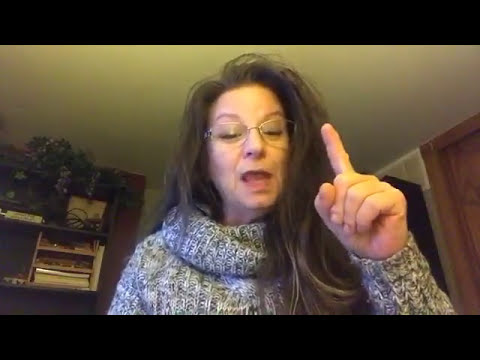The image captures a middle-aged woman in mid-sentence, appearing to be deep in thought while speaking into what is likely a webcam. She is pointing with her left index finger while the other fingers of her left hand are curled into a fist. She has long, slightly messy wavy brown hair with hints of gray, which is draped behind her shoulder on the left side and cascading down on the right. The woman is wearing circular glasses and a thick, gray and white sweater with a large, fluffy turtleneck collar resembling a scarf. Her mouth is partially open as she speaks. In the background, there's a dimly lit room featuring a white ceiling with a yellowish tint from the lighting. Wooden paneling or cabinet doors and a shelf adorned with a green potted plant and a few books can be seen. The setting suggests that she is likely in a home office or living room. The top and bottom of the image have horizontal black stripes, giving it a widescreen appearance.